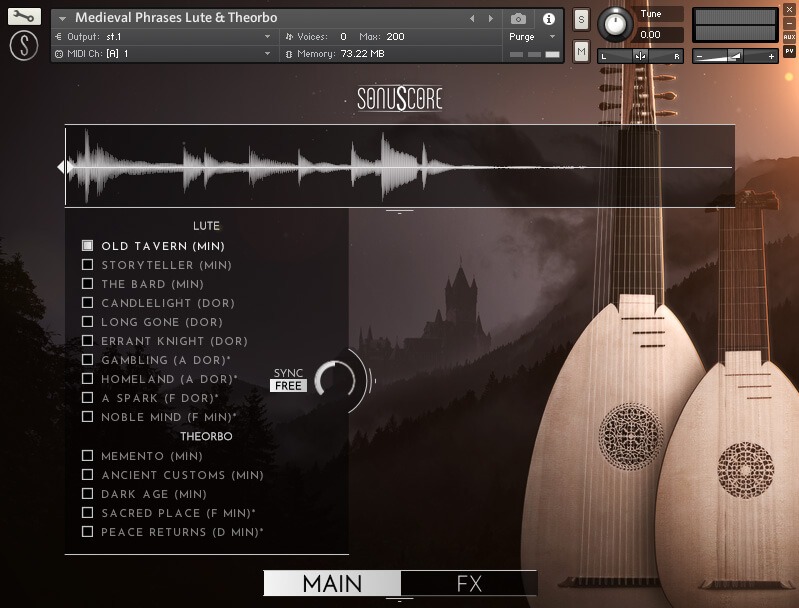The image is a screenshot of a music-related software, displayed in a landscape layout. At the top, the interface features a set of icons, including a wrench and an "S" in a circle, situated in the upper left-hand corner. This is followed by text displaying "SONUSCORE" and another identifying section labeled "Medieval Phrases, Lute, and Turbo." Alongside these, there are icons of a camera, an eye, and indicators for output and memory usage, such as "ST 1 MDI CH a 1 Voice 0 Max 200 0 Memory 73.22 MB."

Below the top section, there is a green-colored musical line, likely representing note strength or musical activity, with the label "SONU SCORE" above it. Underneath this line, there is a comprehensive list of song titles, including "Old Tavern," "Storyteller," "The Bard," "Candle Light," "Long Gone," "Errant Night," "Gambling Homeland," "A Spark," "Noble Mind," "Memento," "Ancient Customs," "Dark Age," "Sacred Place," and "Peace Returns." These songs are displayed with white text against a dark background, each accompanied by checkboxes.

Towards the bottom middle of the screen, there are two buttons labeled "Min" and "FX" in white text. The background of the interface features a castle-like scene with dark hills and some ground area, and prominently showcases two string instruments resembling guitars or mandolins, colored a mix of whitish-brown. This detailed setup implies a medieval, possibly folk, music theme.